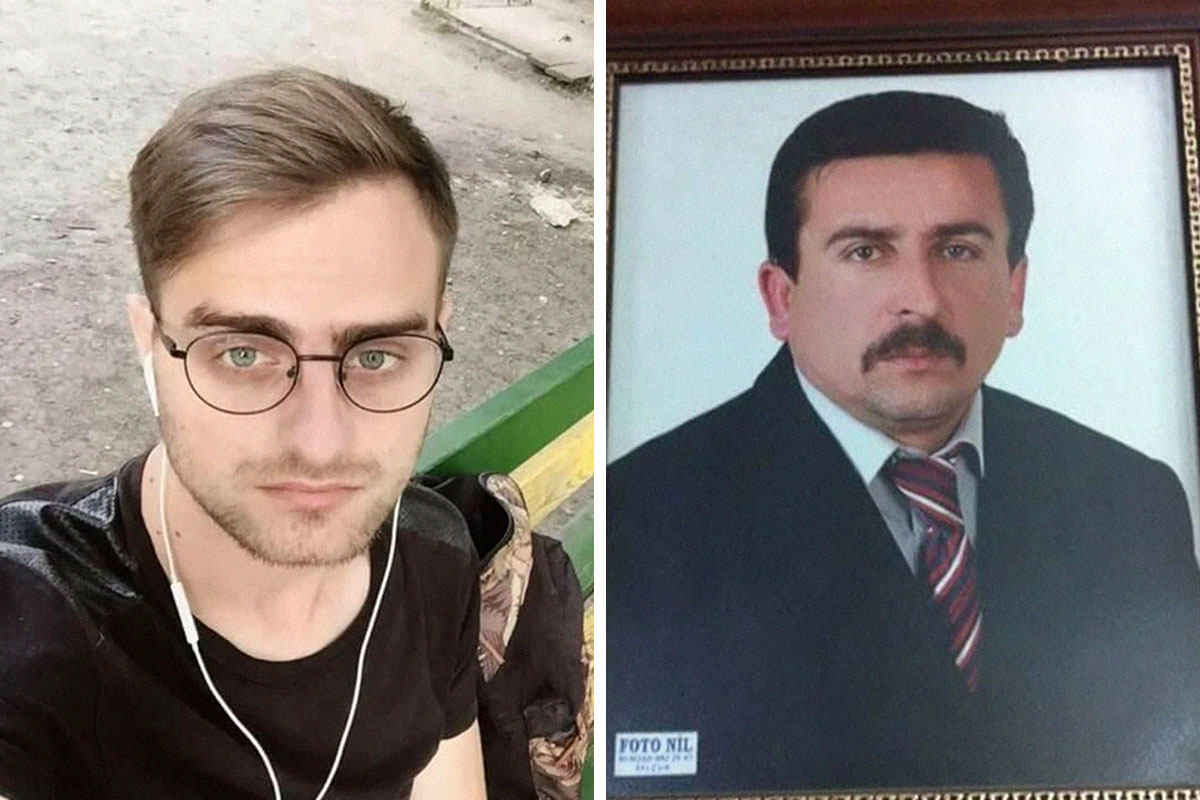The image features two side-by-side photographs of two men who bear a notable familial resemblance. On the left, a younger man possibly in his late 30s to early 40s, with dark brown hair, black wireframe glasses, a scruffy beard, and wired earbuds, stands outdoors. He is dressed casually in a black T-shirt, with a green railing that has a yellow stripe behind him, suggesting he might be on a bridge. His facial expression is solemn as he gazes straight ahead. To the right is an older, formal portrait of another man who appears to be from an earlier era, perhaps the 1970s. This older man has a dark mustache, black hair, and is dressed in a black suit with a white shirt and a red striped tie. The portrait is framed, though only part of the frame is visible. The photograph has the text "FOTONIL" at the bottom left, adding an element of mystery. Both men share similar facial features, indicating they might be related, possibly father and son.